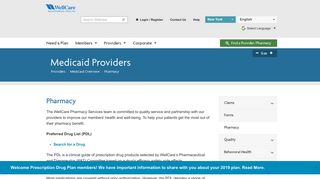The image is a screenshot from a medical website, although the image is notably blurry, making specific details hard to discern. The website seems to be viewed on a desktop or laptop, characterized by a white and blue color scheme predominantly. At the top, there's a gray banner that appears to have "Medicare" written in blue text, though this isn't entirely clear. Beneath this banner are several boxes and drop-down menus, alongside clickable text links such as "Login," "Register," and "Contact Us."

Further down, there's a smaller white banner featuring four clickable drop-down menus, the text of which is unreadable due to the blurriness. Adjacent to these menus is a green button with white text that is also indeterminate. Below this section, a large blue banner prominently displays the text "Medicaid Providers" in white. The rest of the webpage's main content area is white with primarily black text. At the top of this section, "Pharmacy" is written in blue text, followed by several lines of black text that unfortunately cannot be read.